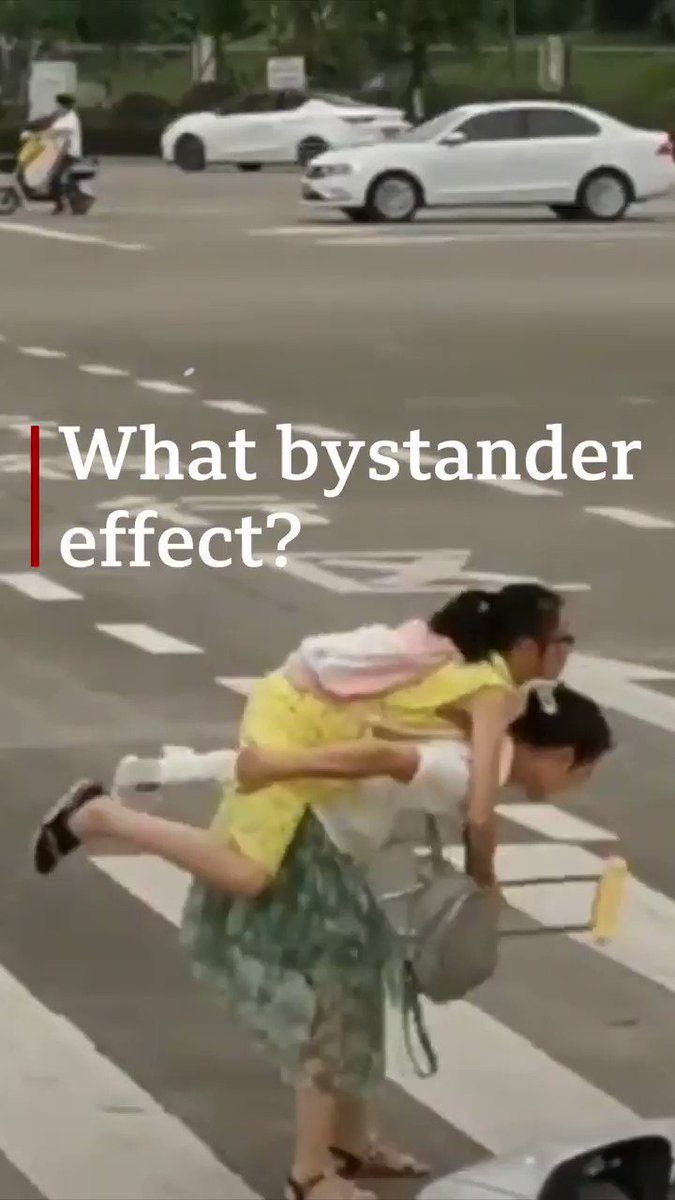The meme is a portrait-oriented photo capturing an urban crosswalk scene. In the foreground, two Asian women are crossing the street. The older woman, with her hair pulled back in a white ribbon, is wearing a short-sleeve white blouse, a greenish-white lace skirt, and brown sandals. She is leaning forward, carrying a younger woman on her back. The younger woman, possibly a teenager, is dressed in a yellow romper and a pink backpack, her hair also pulled back, wearing glasses. She has a black sneaker on one foot, while the other leg is in a white cast, and she's holding a crutch. The background features two white cars—one parked and one possibly moving—and a man in a white shirt riding a motor scooter. Further behind, there's a fence, some grass, trees, and indistinct signs. Above the women, text in white serif font reads, "What bystander effect?" separated by a vertical red line, reinforcing the meme's inquiry about the bystander effect.